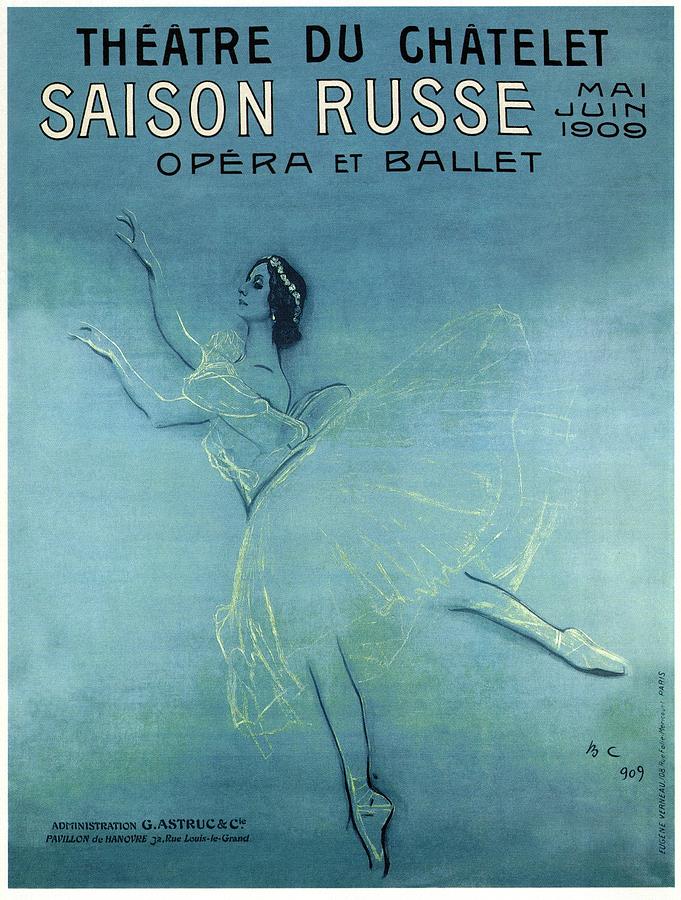This image is a detailed, color illustration in portrait orientation, serving as the vintage cover of a 1909 ballet and opera program from the Théâtre du Châtelet in Paris. The background is blue, creating a striking contrast with the central figure—a ballerina, who is the primary focus of the illustration. The ballerina is captured mid-air, gracefully floating. Facing the left, she kicks her leg back, her dark hair pulled back and adorned with a floral band. Her arms are elegantly raised forward above her head. She wears a sheer ballet costume top paired with a knee-length tutu skirt and ballet slippers, her pointed feet emphasizing her poised grace. The top of the image features black text "Théâtre du Châtelet," followed by white text "Saint-Saëns-Rousseau." To the right, in black text, are the months "Mai-Juin 1909" and below, "Opéra et Ballet." The bottom left corner contains additional text in black, likely detailing the administration. This vintage pamphlet, with its detailed illustration and classic typography, evokes the elegance and artistic essence of early 20th-century French ballet and opera culture.